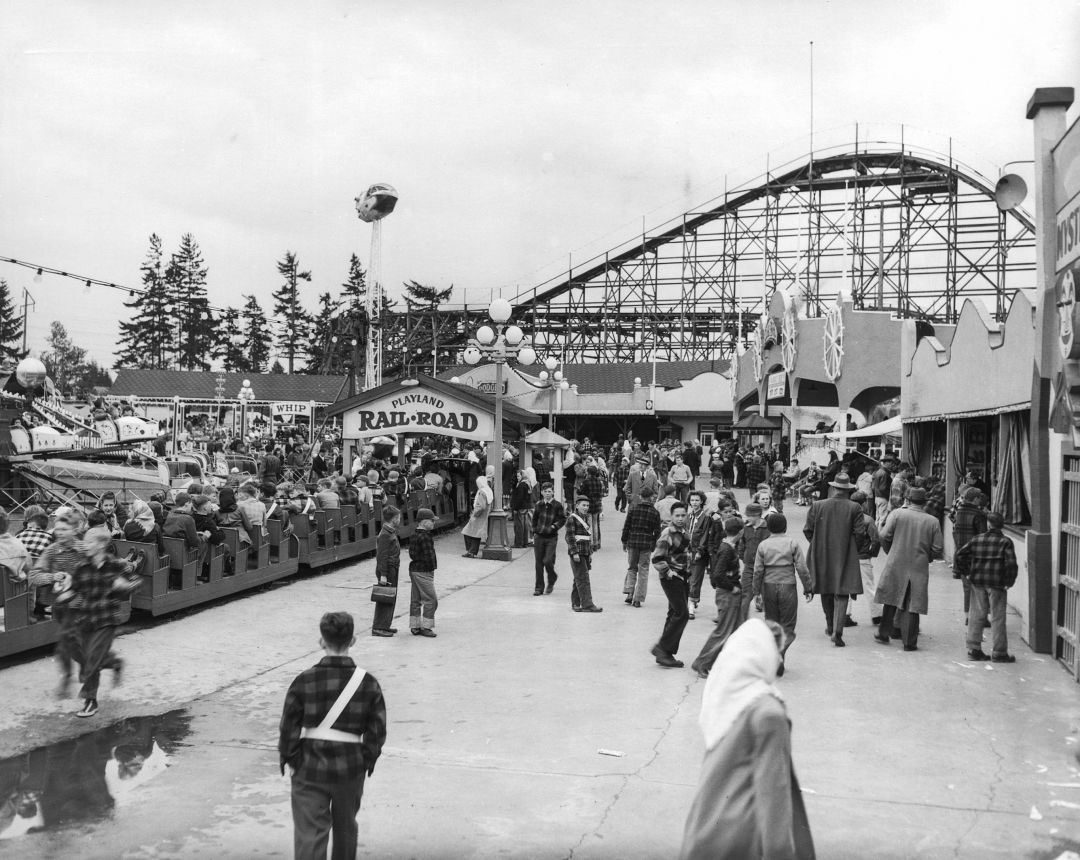This black-and-white photograph captures a bustling scene at an amusement park, likely from the 1930s or 1940s, characterized by its nostalgic charm. Dominating the background is an imposing roller coaster with intricate scaffolding. The foreground is alive with activity, centered around the Playland Railroad—a quaint ride featuring small railroad cars fully occupied by eager passengers. To the left of this ride, there's a spinning attraction for children. The scene is set on a concrete walkway, surrounded by various booths and facades of midway games and attractions. The crowd is a mix of men in top hats and long coats, women in long dresses and headscarves, and numerous boys in plaid long-sleeve shirts, some appearing to serve as staff with safety belts around their waists. The sky is a moody gray, adding a timeless atmosphere to this lively snapshot of mid-20th century amusement park life.